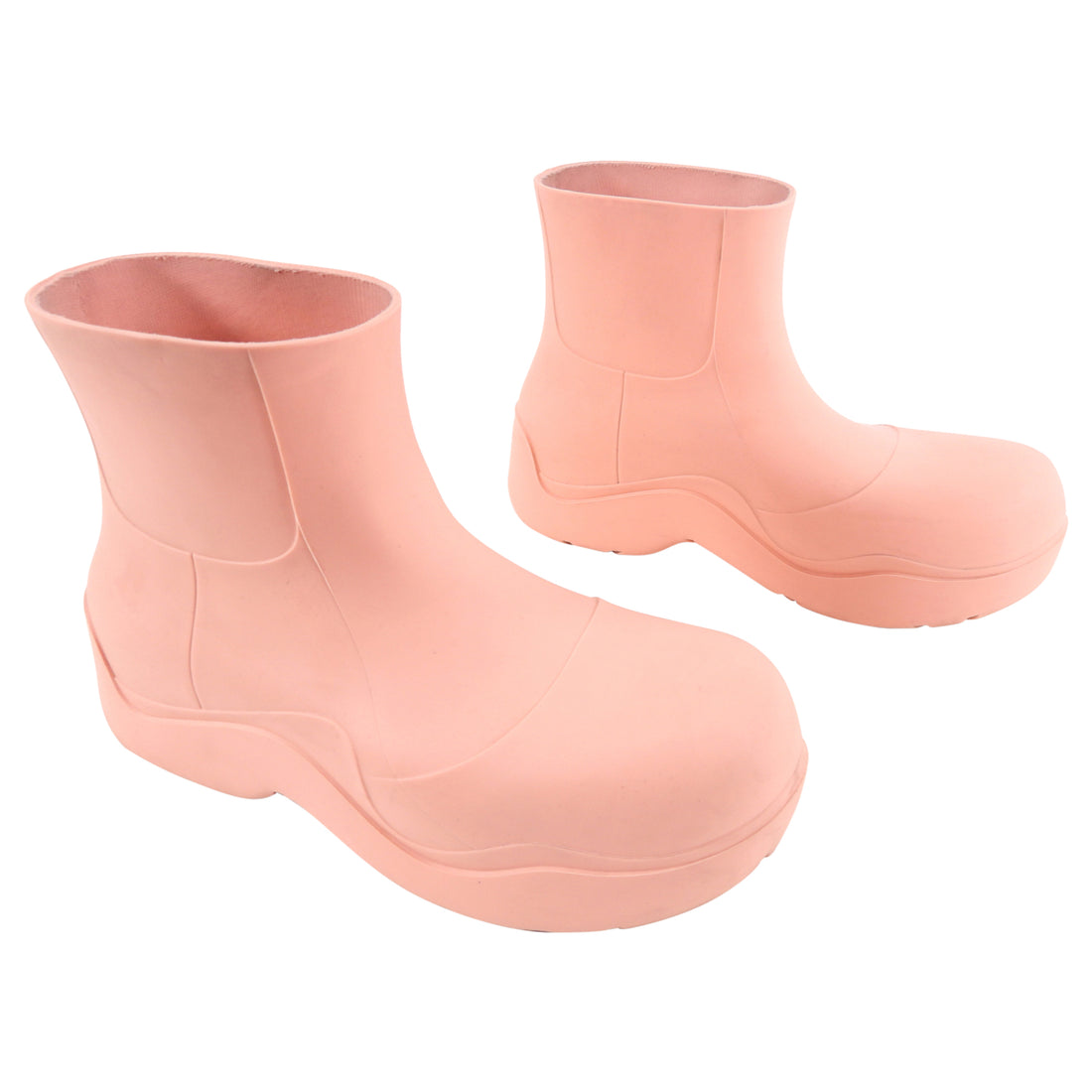This image depicts a pair of pink children's rain boots set against a featureless white background. The boots have a distinctive, slightly rounded and blunt toe shape, reminiscent of Crocs but without any holes or openings. They are crafted in a light peachy blush color and rise just above the ankles, similar to Chuck Taylor's sneakers. The entire surface features grooves that suggest they were made by a 3D printer or similar plastic extrusion process. These boots also have deep, thick soles with hints of light tread along the bottom, and the soles extend slightly up the heel, providing additional support. There may be elastic around the top for a better fit, though this detail is not confirmed.